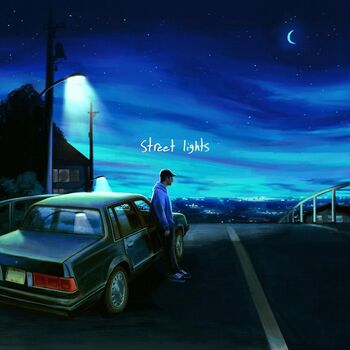The album cover titled "Streetlights" features a detailed drawing of a young man in a blue hoodie and baseball cap, leaning against a boxy 1980 sedan parked on the side of a street. The street is a curved road, possibly a bridge, with railings on both sides and a white line in the middle. Above, the sky transitions from light blue at the horizon to dark black at the top, adorned with a crescent moon and scattered stars. Two streetlights illuminate the scene, one of which casts a glow directly over the car. A cityscape with twinkling lights stretches out below the hill, while a silhouetted house with lit windows and a telephone pole can be seen on the left. The title "Streetlights" is prominently displayed, capturing the nighttime ambiance and reflective mood of the setting.